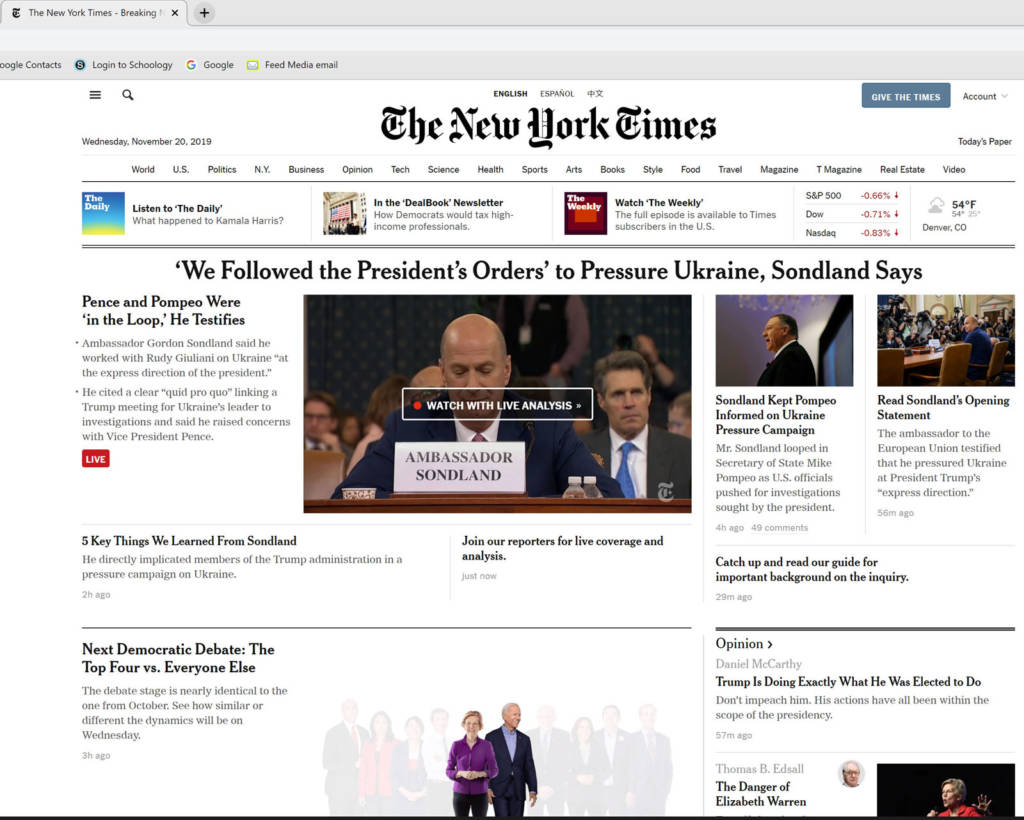A detailed and cleaned-up caption for the described image could be:

"A screenshot of the New York Times website from Wednesday, November 20th, 2019. The New York Times title is prominently displayed at the top left of the page, alongside the date. Below the title is a comprehensive menu offering various sections such as ‘World,’ ‘U.S. Politics,’ and more. At the top of the page, there are links to audio programs, including 'Listen to The Daily' and 'Watch The Weekly,' as well as the DealBook newsletter. To the right, important financial information is displayed, featuring the performance of three major markets and the current weather.

Centrally positioned is the main headline of the day: 'We Followed the President's Orders to Pressure Ukraine, Sondland Says.' To the left of this headline, a secondary highlight reads: 'Pence and Pompeo Were in the Loop, He Testifies.' On the right side, further details are provided, stating: 'Sondland Kept Pompeo Informed on Ukraine Pressure Campaign,' accompanied by a link to 'Read Sondland's Opening Statement.'"